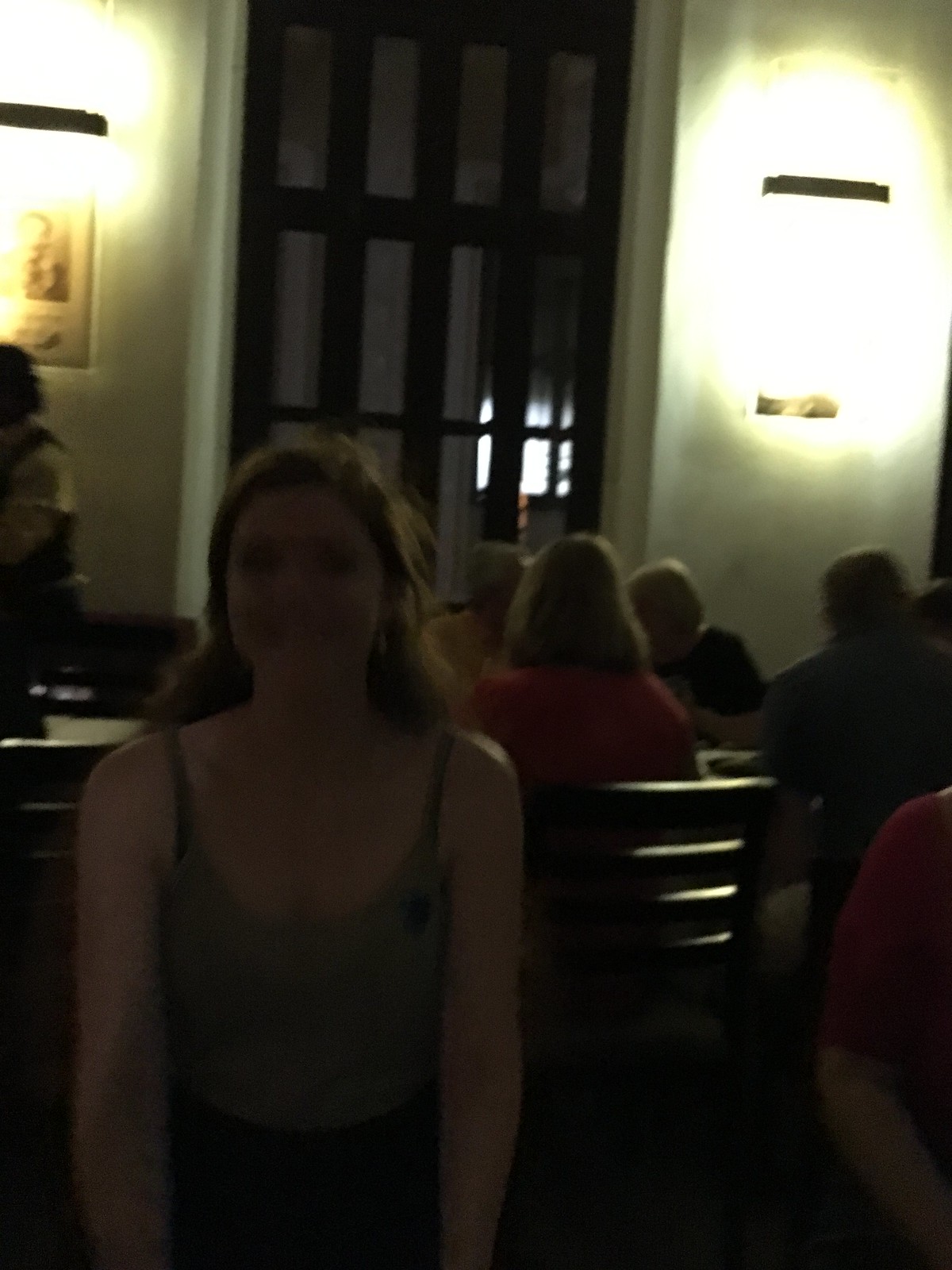In this cozy indoor photo, we are positioned inside someone's home. The setting features a wooden door with elegant glass panes, adding a touch of warmth to the interior. In the background, an inviting scene unfolds: a table around which people are gathered, absorbed in conversation. A charming sconce light mounted on the wall gently illuminates the area.

In the foreground, a young lady takes center stage, dressed in either black pants or a skirt paired with a gray tank top that has a small pin adorning the front. Her dark hair cascades down as she stands slightly blurred, with her face not entirely in focus, and she faces away from the light source. Beside her, an individual in a red short-sleeve shirt adds a burst of color to the scene. 

The background features more figures; a woman clad in red sits next to a man wearing blue, although the details of the other people at the table are less discernible due to their positioning and the focus of the camera. The overall ambiance is intimate and homey, capturing a candid moment of everyday life.